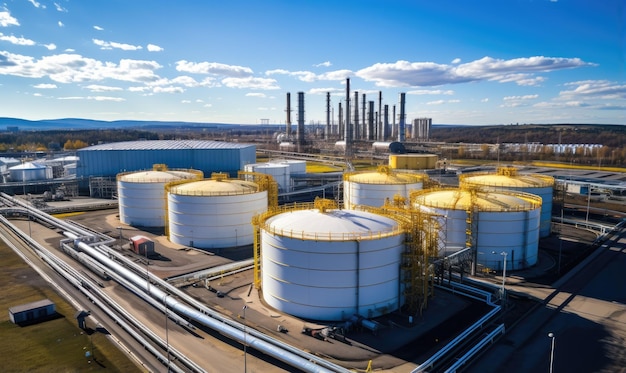This photograph captures an expansive industrial facility, likely an oil refinery or large-scale manufacturing plant, viewed from an elevated perspective. Dominating the foreground are several enormous white cylindrical tanks—five or six in total—each fitted with yellow railings circling the tops and yellow ladders affixed to their sides for access. These tanks are surrounded by a network of metal pipes and connected to adjoining structures. In the middle ground and stretching into the distance, towering smokestacks—approximately 15 in number—pierce the sky, asserting the industrial nature of the setting. 

To the left of the frame, a sizable, tin-like building adds to the industrial complexity. The backdrop features a deep blue sky dotted with scattered, fluffy white clouds, all under the bright daylight. The horizon is adorned with gentle hills and an array of trees, setting a natural scene against the industrial foreground. A road curves around the tanks, and some areas of bare ground can be seen, emphasizing the functional and utilitarian layout of the facility. The image is rich in detail and depth, offering a clear and comprehensive view of this extensive industrial environment.